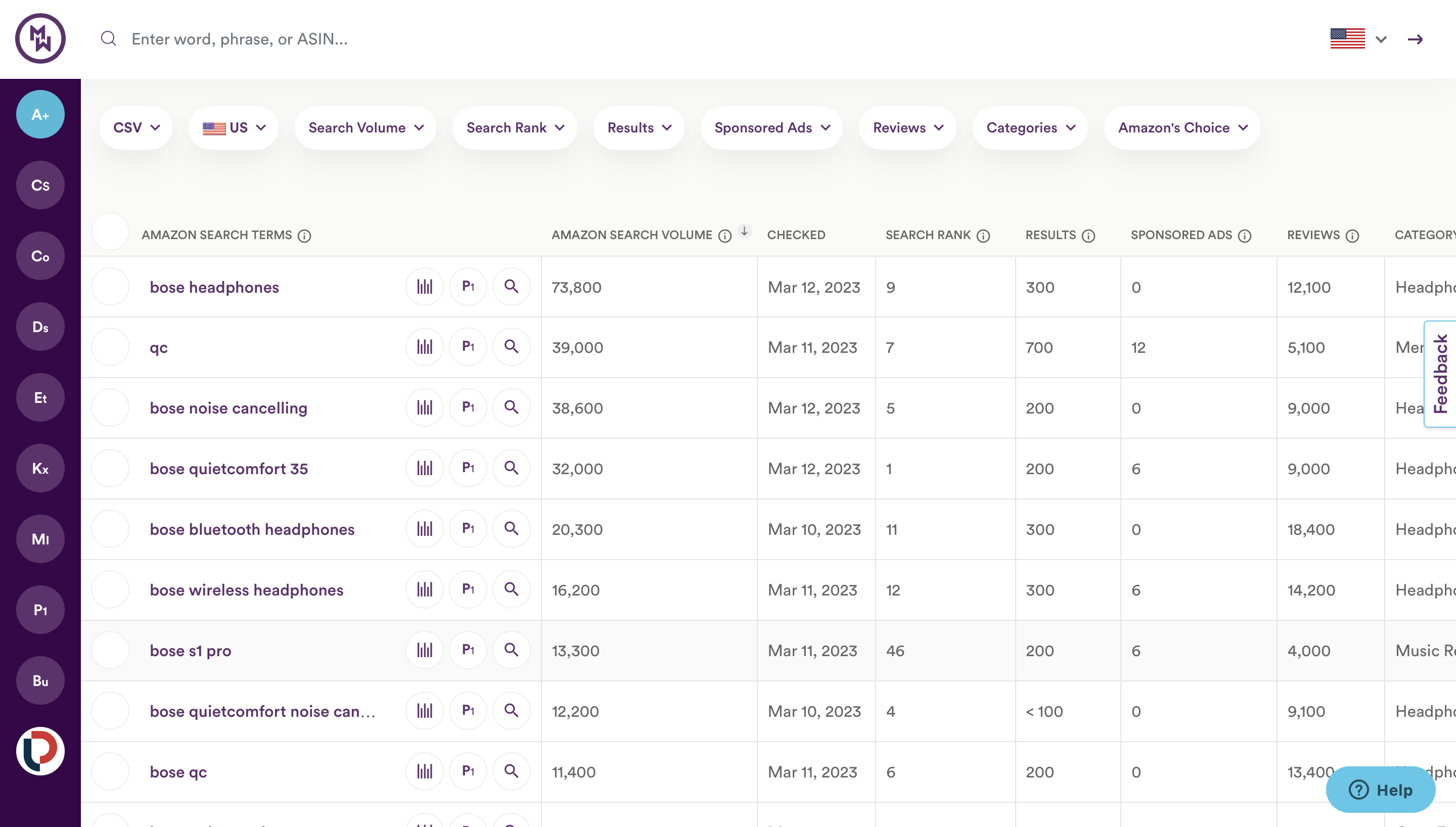The image depicts a detailed interface for a website designed to analyze and display keyword performance metrics for Amazon. The website features a predominantly purple and white color scheme and organizes the information in a well-structured chart.

At the top of the interface, there is a white circle with a purple border, displaying a purple "M" and an inverted purple "M" beside it. To the right, an American flag icon signals the site's current country setting, accompanied by a drop-down arrow for changing the country. Below this is a purple arrow icon.

Centrally located is a search bar labeled "Enter word, phrase, or ASIN" with a magnifying glass icon, allowing users to input their search terms. On the left-hand side, a vertical purple box features a series of circles, each containing white lettering except for the top one, which is light blue with "A+" inscribed in white. The other circles, all purple with white letters, are labeled respectively: CS, CO, DS, ET, KX, ML, P1, and BU. A white circle with intersecting red and black lines that resemble the letter "P" is also present.

The top menu includes options labeled CSV, country (US selected), search volume, search rank, results, sponsored ads, reviews, categories, and Amazon's Choice, each featuring a drop-down arrow for further customization.

Beneath the top menu, the interface showcases key metrics including Amazon search terms, Amazon search volume (checked), search rank, results, sponsored ads, reviews, and categories. Additionally, there are options for "help," highlighted in blue, and "feedback," highlighted in purple.